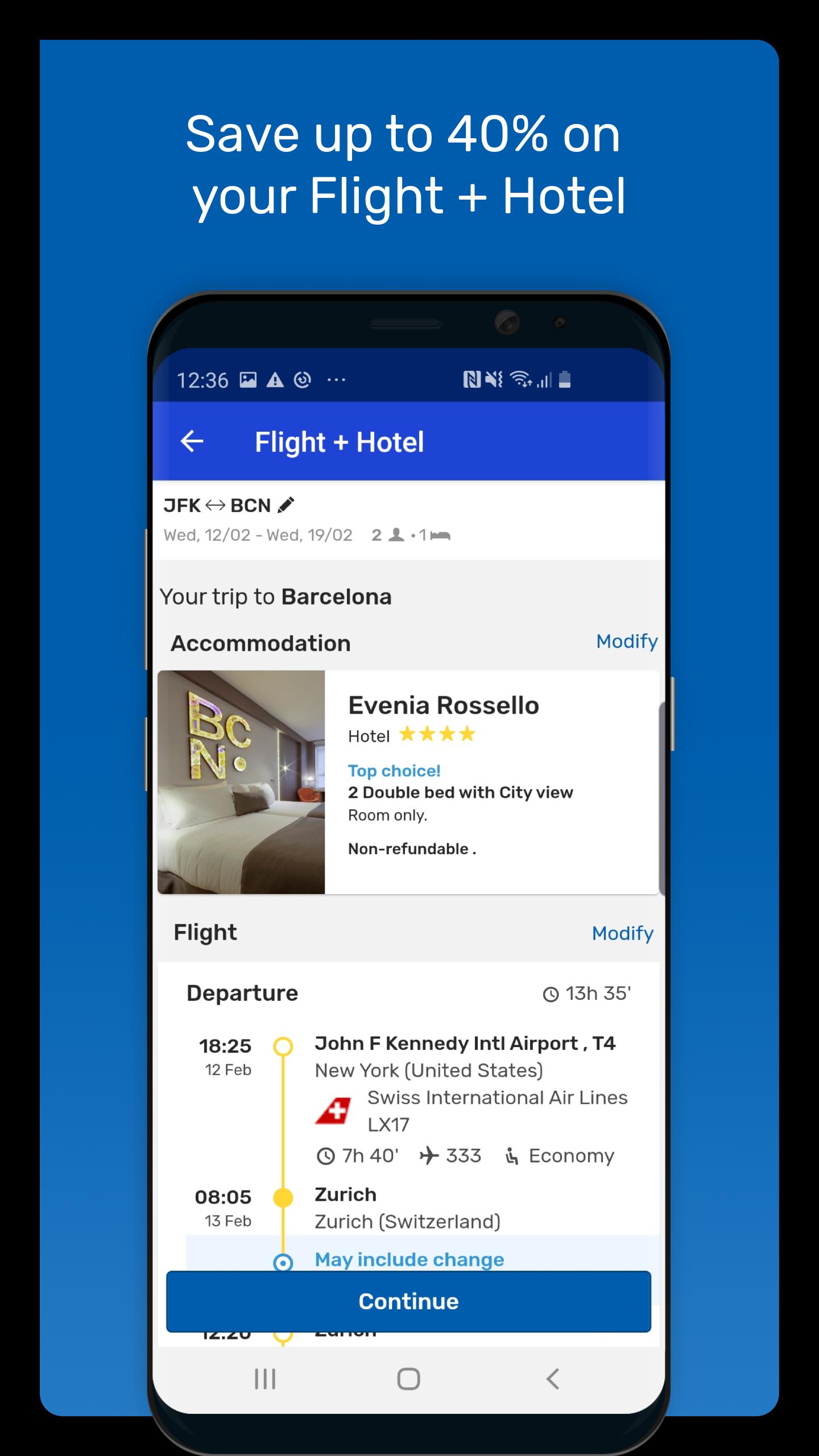**Detailed Descriptive Caption for Image:**

"Travel Advertisement: Save up to 40% on PCP plans including hotels. The image prominently features various travel-related icons and symbols. 

1. **Visual Elements:**
   - A triangular icon displaying '1236'.
   - An NFC speaker with a slash through it, indicating 'no NFC'.
   - Full WiFi signal with almost full bars.

2. **Battery and Safety:**
   - A moment of safety battery icon, showing a blue bar towards the right.
   - Adjacent text indicating battery safety levels.

3. **Navigation and Airport Codes:**
   - Left and right arrows indicating navigation.
   - Airport codes: JFK (New York), BCN (Barcelona).

4. **Accommodation Details:**
   - Wednesday: Dates are shown as 12/02 and 19/02.
   - Room info: 2 people, 1 bedroom, 1 bed.
   - Description: "New traits of Barcelona accommodation," featuring Hotel Eviania Rosella.
   - Hotel rating: 1234, gold stars, 'Top Choice'.
   - Room type: Twin double bed with city view, room only, non-informable.

5. **Visual and Textual Elements:**
   - A picture of a lens.
   - Bed with letters on the wall.

6. **Flight Information:**
   - Modified departure times: 13 hours 35 minutes, 18:25.
   - Airports: New York (JFK), Kansas, Zurich (Swiss), Switzerland (Zurich Airport, LX17).
   - Flight duration: 7 hours 40 minutes.
   - Seating: Window seat, 333.
   - Flight class: Economy, flight number 535.
   - Trend reference: Canadian industrial airport total footprint is 2400 units.

7. **UI Elements:**
   - A blue rectangle button labeled 'Continue'.
   - Bottom left displays a numeric sequence: 1, 2, 3 square.
   - Bottom right features a navigation arrow pointing left.
   - Smartphone icon depicted.

Overall, the image serves to promote travel packages combining flight and hotel bookings with significant discounts and provides detailed travel and accommodation options."